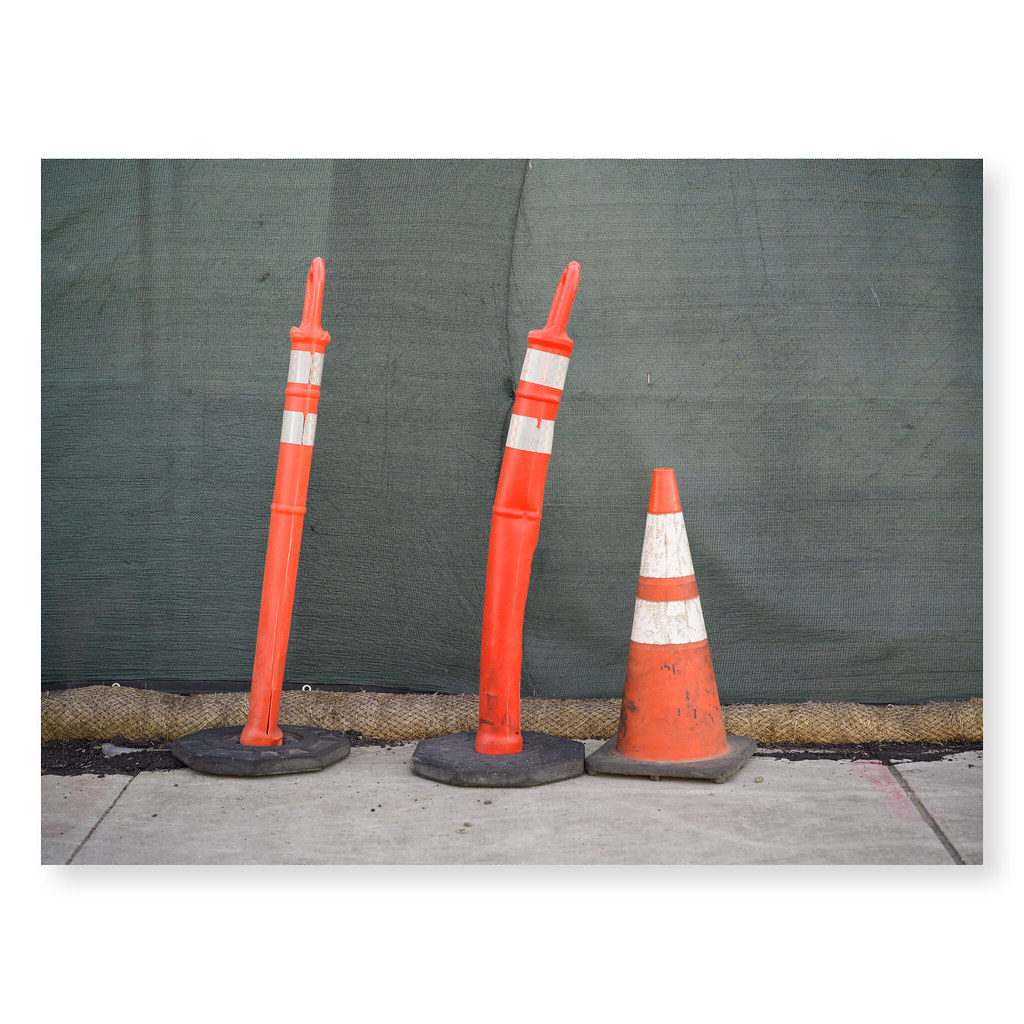In this outdoor color photograph, three distinct traffic markers are prominently displayed on a concrete sidewalk. Positioned from right to left, the first marker is an orange traffic cone with a black square base and two white horizontal stripes near its top. Next to it, there are two cylindrical traffic markers with black round bases, each featuring two white horizontal bands at the top and an orange ring. The sidewalk shows signs of recent construction, as evidenced by some blacktop spilled beside the leftmost marker. In the background, a black mesh netting is stretched against a chain-link fence, partially covered by a green camouflaged tarp that extends to where it meets the cement surface.